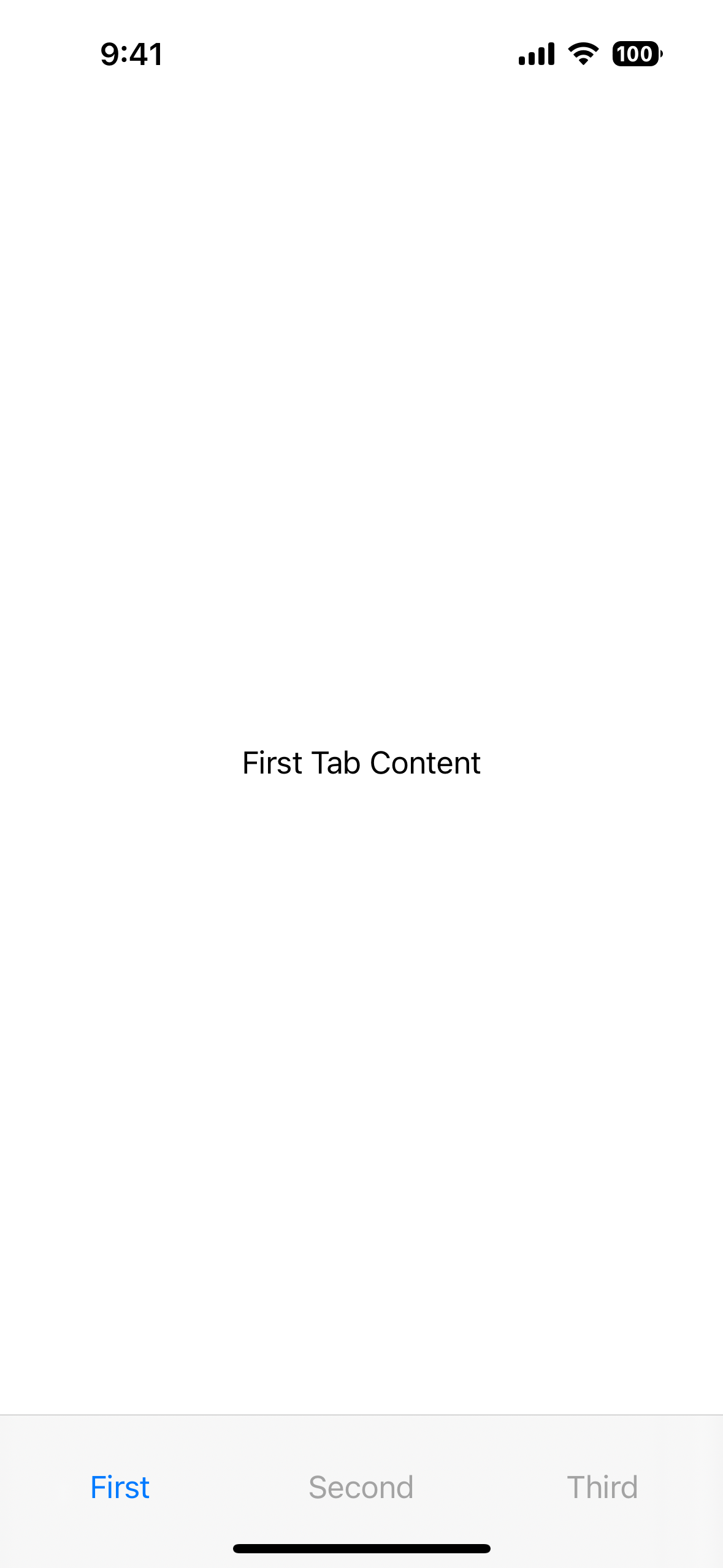The image depicts the screen of an Apple smartphone displaying the time 9:41 in the top left corner. In the top right corner, three black icons can be seen: a fully charged battery, Wi-Fi signal, and network signal. The central part of the screen displays text that reads "First tab content" in black on a white background. At the bottom of the screen are three tabs. The first tab on the left is highlighted in blue, indicating it has been selected. The text "First tab content" is also repeated in the center of the screen, confirming the selection. The second tab is in the middle, and the third tab is on the right. The background of the three tabs is a light gray color, while the inactive tabs are colored in a plain gray. Additionally, a black minimize slider is visible at the very bottom of the screen. The overall background of the image is predominantly white, except for the tab area at the bottom.